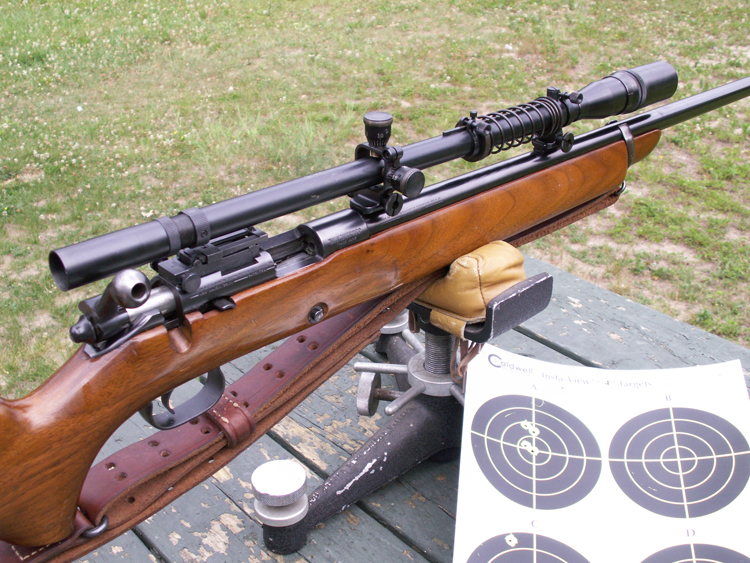The photograph captures a scene at a shooting range featuring a wooden rifle mounted on a sturdy black tripod, which is attached to a weathered wooden table. This table appears to have been painted gray or blue but has since become weather-beaten, exposing patches of the underlying wood. Located in a flat, grassy field, the vibrant green grass surrounds the setup, contrasting with the rustic aesthetic of the table.

The rifle itself, crafted from medium-stained wood with a somewhat shiny finish, showcases a long black barrel and trigger, complemented by an extended, thin metal scope. The scope includes a prominent lens toward the front, backed by a spring mechanism. A leather strap, neatly tied with a leather tie to stay out of the way, hangs beneath the rifle.

Resting on the table beside the tripod is a white target paper laid out in a 2x2 grid format with circular targets. The top-left target on the page displays four bullet holes, with two hitting the bullseye and two within the ring just above it. This meticulous arrangement suggests a shooter making precise shots, aided by the stability provided by the mounted setup.